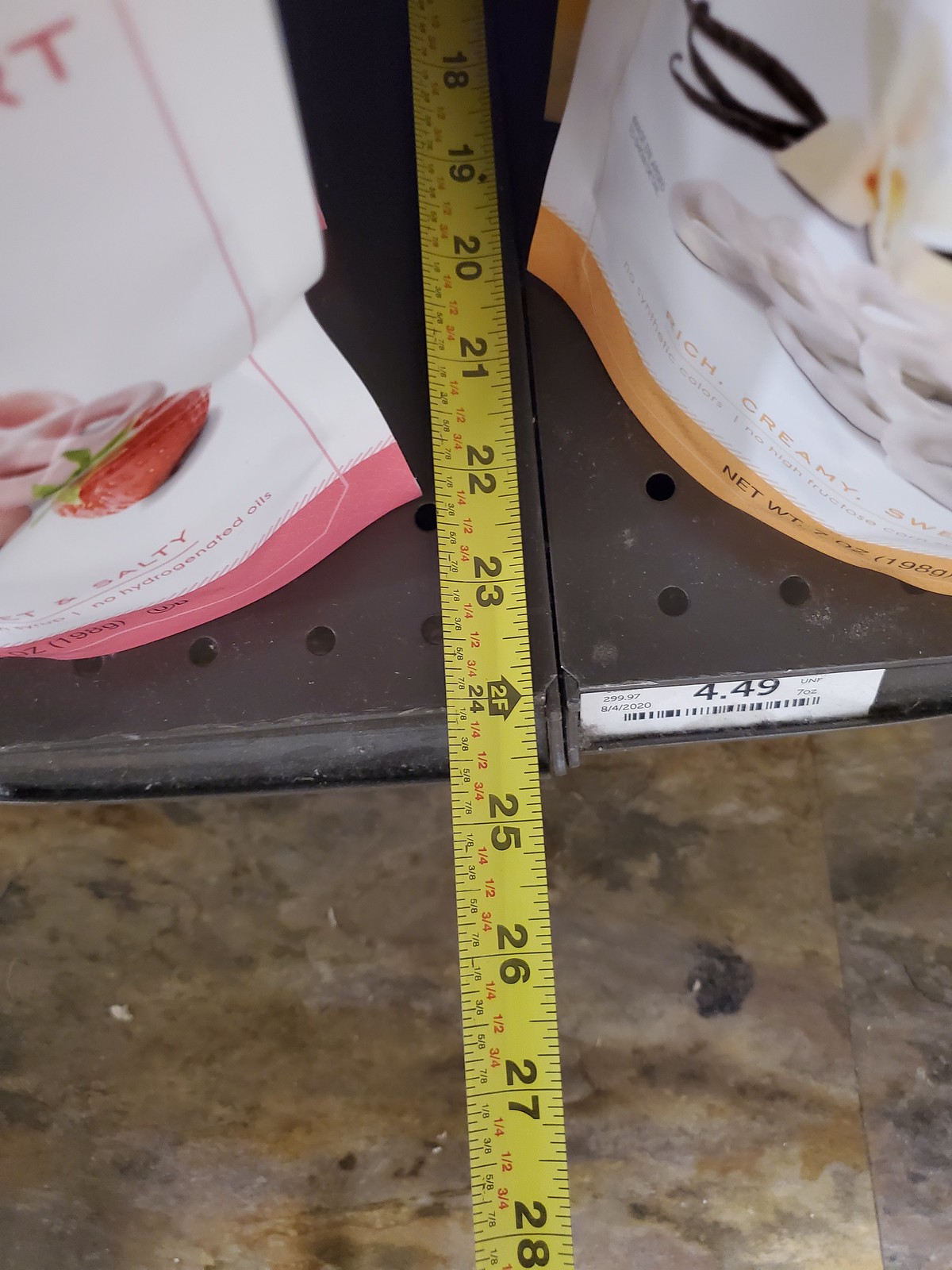In the photograph, there is a close-up view of a shelf featuring several items. Dominating the image is a yellow tape measure in the center. The tape measure displays large graduation marks and figures ranging from 18 to 28, with smaller increments between them. 

To the left of the tape measure, there is a white packet with pink linings and a pink bottom section, featuring an outline of a strawberry, suggesting that it might be an edible product. To the right, another white packet with similar pink accents is visible, though the text on it is difficult to read due to the angle of the shot.

At the bottom right corner of the shelf, a white paper is affixed, showing a price of $4.49 along with barcodes printed in black. This detailed composition provides a clear view of the items and price on display.